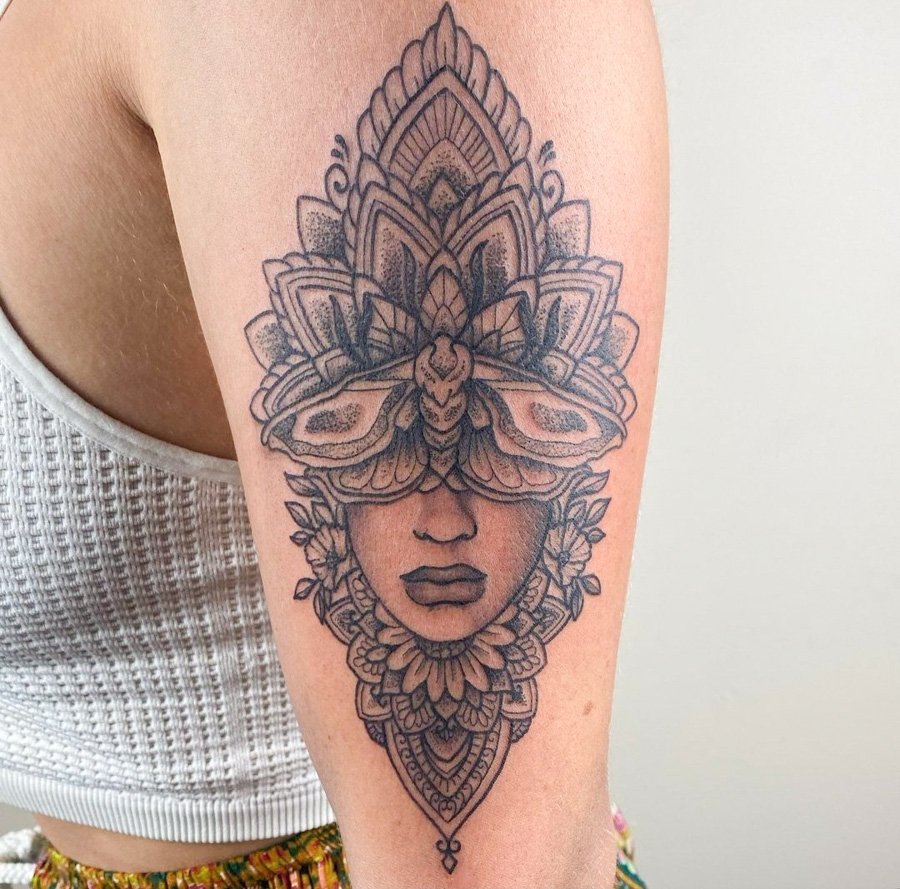The photograph captures a close-up of a light-skinned woman's left arm, showcasing a freshly done, intricate, black and white tattoo. Her arm is positioned centrally, framed against a plain white wall. She wears a white woven crop top, and the rim of this top is just visible alongside her multicolored, yellow and gold patterned pants. The tattoo spans from just below her shoulder to her elbow, featuring a striking artistic rendition. The design includes the lower half of a woman's face with visible nose and lips, while a detailed moth with open wings obscures her eyes. Surrounding this central image, the tattoo incorporates a headdress with leaf and water splash designs, as well as additional floral and leaf motifs that taper towards the bottom, creating a beautifully elaborate and flowing aesthetic.